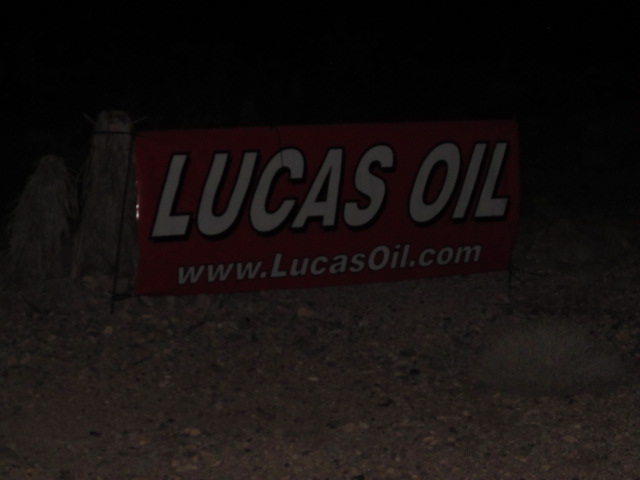In this very dark photograph, the central focus is a prominent red rectangular Lucas Oil sign. The sign, which appears to be affixed to black metal poles, displays the text "LUCAS OIL" in large white block letters with a black outline. Beneath this, the website "www.lucasoil.com" is written in white letters with a similar black outline. To the left of the sign, there is a visible post or stone pillar, suggesting the sign is attached to it. The foreground reveals rocky soil with a few larger stones and a small shrub in the lower right-hand corner. The surrounding environment, including the area above and to the right of the sign, is enveloped in darkness, indicating the photo was taken at night.